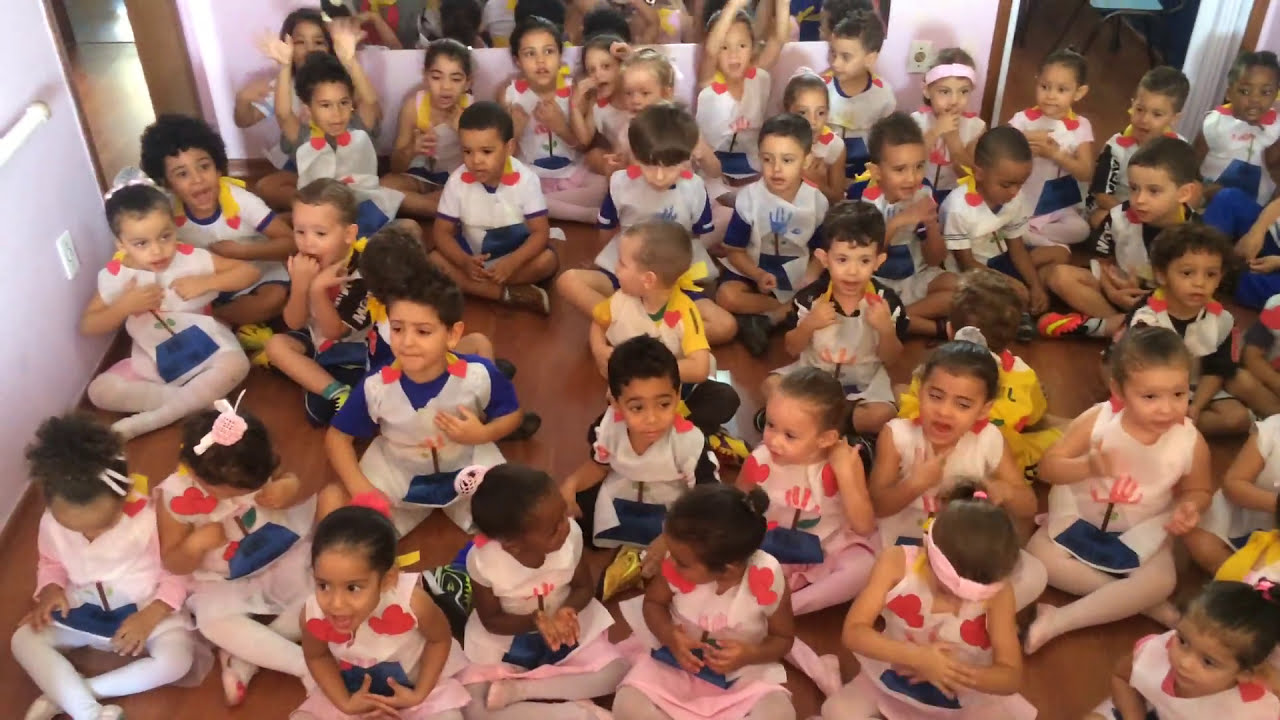This is a captivating photograph of approximately 20 school-aged children, ranging from about five to eight years old, seated cross-legged on a wooden floor in a vibrant, colorful room, likely a classroom or play area. The diverse group of children, featuring boys and girls of various ethnicities including African, Caucasian, Asian, and Hispanic descent, are all dressed in unique white outfits adorned with red heart designs and some with hints of yellow and orange. In the front row, three girls are notably positioned: one potentially of Amerasian or Hispanic descent, another of African descent, and a third with dark skin and hair pulled back in a bun, whose ethnicity is not immediately clear. A fourth girl, appearing Caucasian, bows her head with her arms crossed. The children display a variety of expressions, some smiling or laughing, and others deep in conversation or in playful gestures, enhancing the sense of liveliness and excitement in the image. Behind them, the background features a mirror at the center top, a door on the top right, and a pink wall with a white railing on the top left, adding depth and a lively context to the scene, indicating an engaging moment in what could be a rehearsal or playful activity.